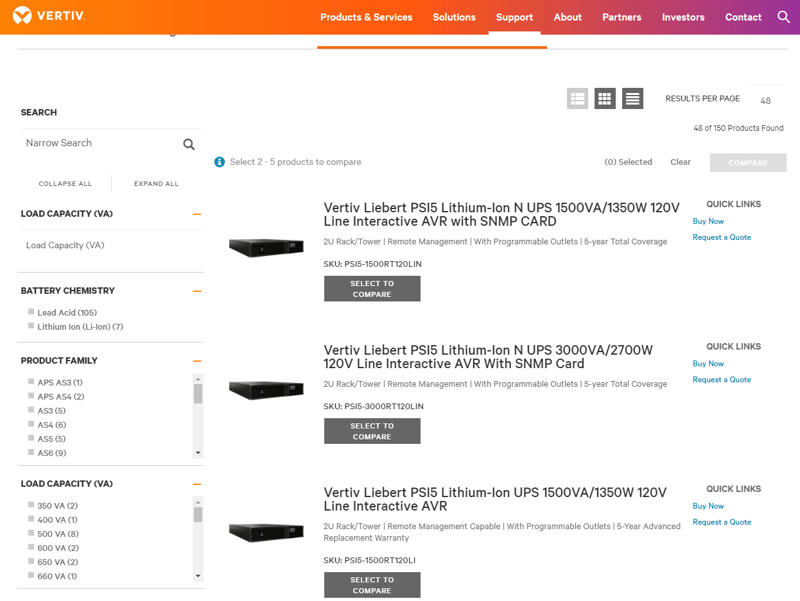This image depicts a web page from Vertiv, a company specializing in critical infrastructure. The banner at the top showcases a gradient transitioning from orange to purple, creating a vibrant and engaging visual effect. On the left side of the banner, the company's name, "VERTIV," is prominently displayed in uppercase letters, while the right side features an organized navigation menu. The menu includes links labeled as Products & Services, Solutions, Support, About, Partners, Investor, and Contact, accompanied by a search icon.

Beneath this colorful banner, the content is neatly presented with black or blue text set against a clean white background. The blue text is used selectively, running down the right side of the page, highlighting options such as "Buy Now" and "Request a Quote." These are presumably calls to action for potential customers.

The main section of the page is dedicated to showcasing UPS (Uninterruptible Power Supply) products. Three specific products are listed, starting with the "Vertiv Liebert PS15 Lithium-Ion UPS." Each product description includes detailed technical specifications crucial for informed decision-making.

To aid users in refining their search, a column on the left side of the content offers various filtering options. These filters allow users to narrow down the product options based on criteria such as load capacity, battery chemistry, product family, and more, ensuring they can find the most suitable product for their needs.